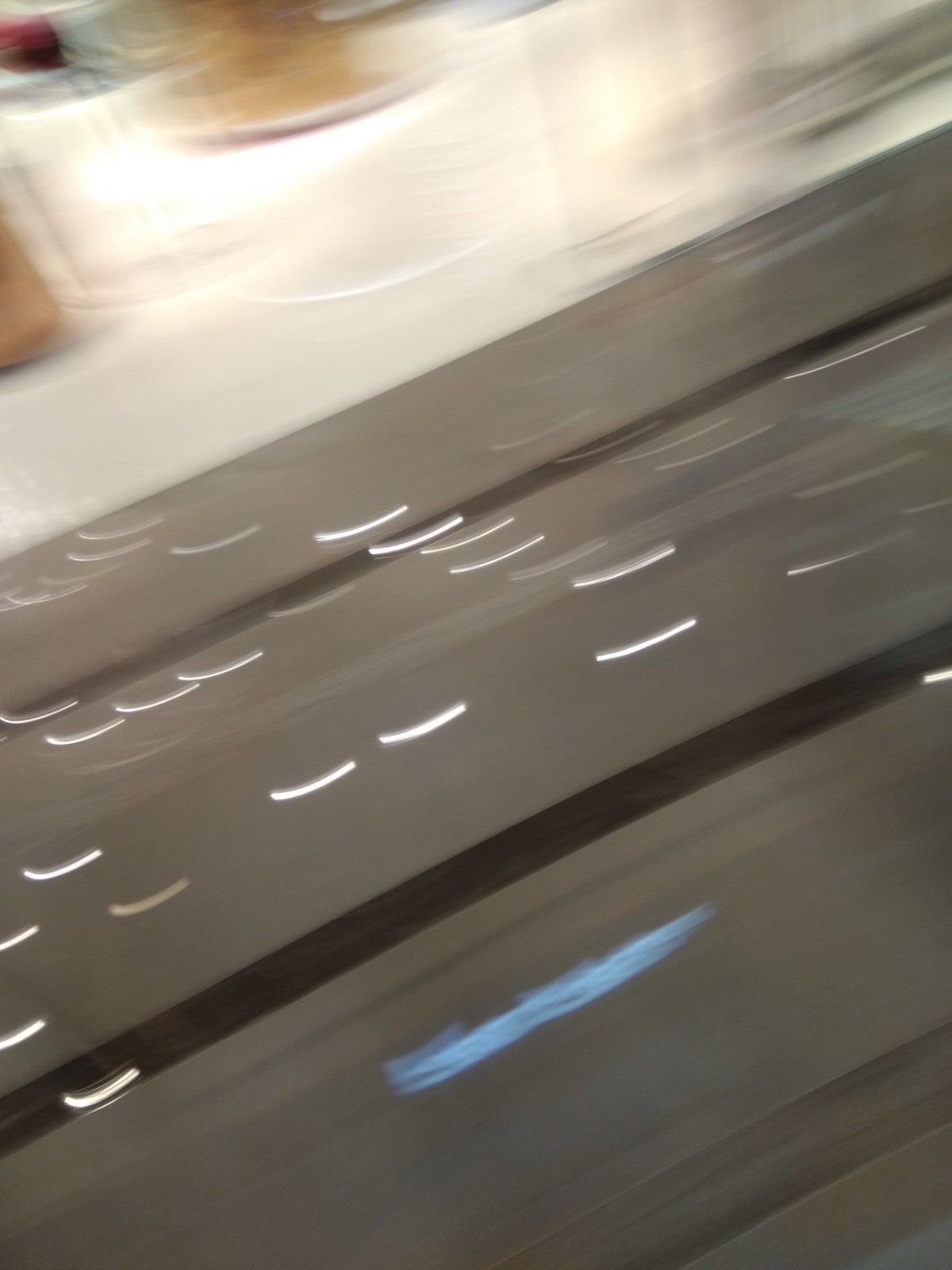This image is characterized by its low quality and motion blur, making it difficult to discern specific details. In the bottom middle section, there's a light blue object whose exact nature is unclear due to the blurriness. The background is predominantly gray, bisected by a black horizontal line that stretches from the bottom left to the right edge of the frame. Above this black line, there are several white lines, the purpose of which is indeterminate. In the top left corner, there is a white object that appears to be made of plastic. Overall, the image's fuzziness and low resolution significantly obscure its content.